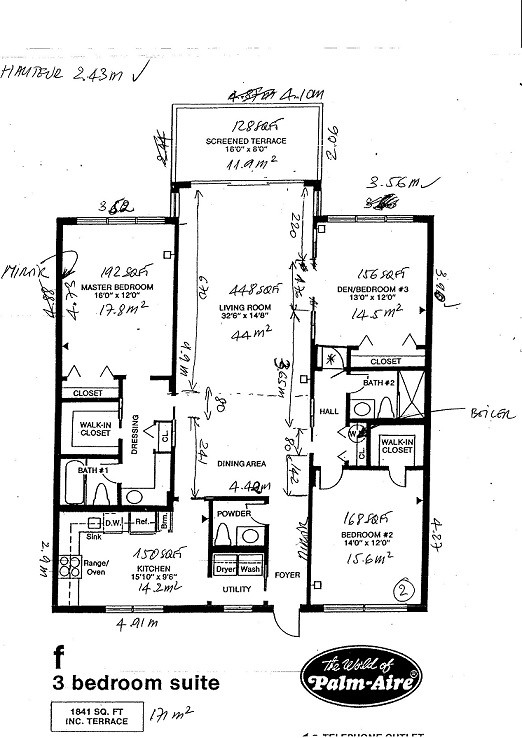**Caption:**

This intricate blueprint photograph showcases the detailed floor plan of a luxurious three-bedroom suite spanning 1,841 square feet, inclusive of a terrace—a total area of approximately 171 square meters. The image is densely populated with various types of writing, including cursive and light-brushed white text. At the top of the blueprint, prominently highlighted within an oval with a black background, the phrase "The World of Palm Aire" stands out, with "the world of" rendered in cursive and "Palm Aire" in a distinct, elegant white script.

The floor plan provides a comprehensive layout of the suite, including:

- A **master bedroom** measuring 16 by 12 feet, located on the left side of the plan. Adjacent to it is a **large walk-in closet** and a **dressing area**, along with **bath number one** directly underneath.
- A **spacious living room** with dimensions of 32 by 14 feet, offering ample space for relaxation and entertainment.
- A **kitchen** positioned below the master bedroom, extending to 16 feet in length.
- On the right side, there is a **powder room**, a **laundry area** with designated spots for a dryer and washer, and a **utility room**.
- Above the kitchen area, the plan features a **dining area** that seamlessly connects to the living room.
- To the right of the dining area, a **den** and **bedroom number three** are situated, with a **closet** between them and **bathroom number two**.
- A **hallway** at the bottom right leads to **bedroom number two**, which is complemented by a **walk-in closet** nestled between the bedroom and **bath number two**.

Each room and utility space is carefully labeled, reflecting a well-thought-out design that maximizes the available space and highlights the suite's luxurious amenities.